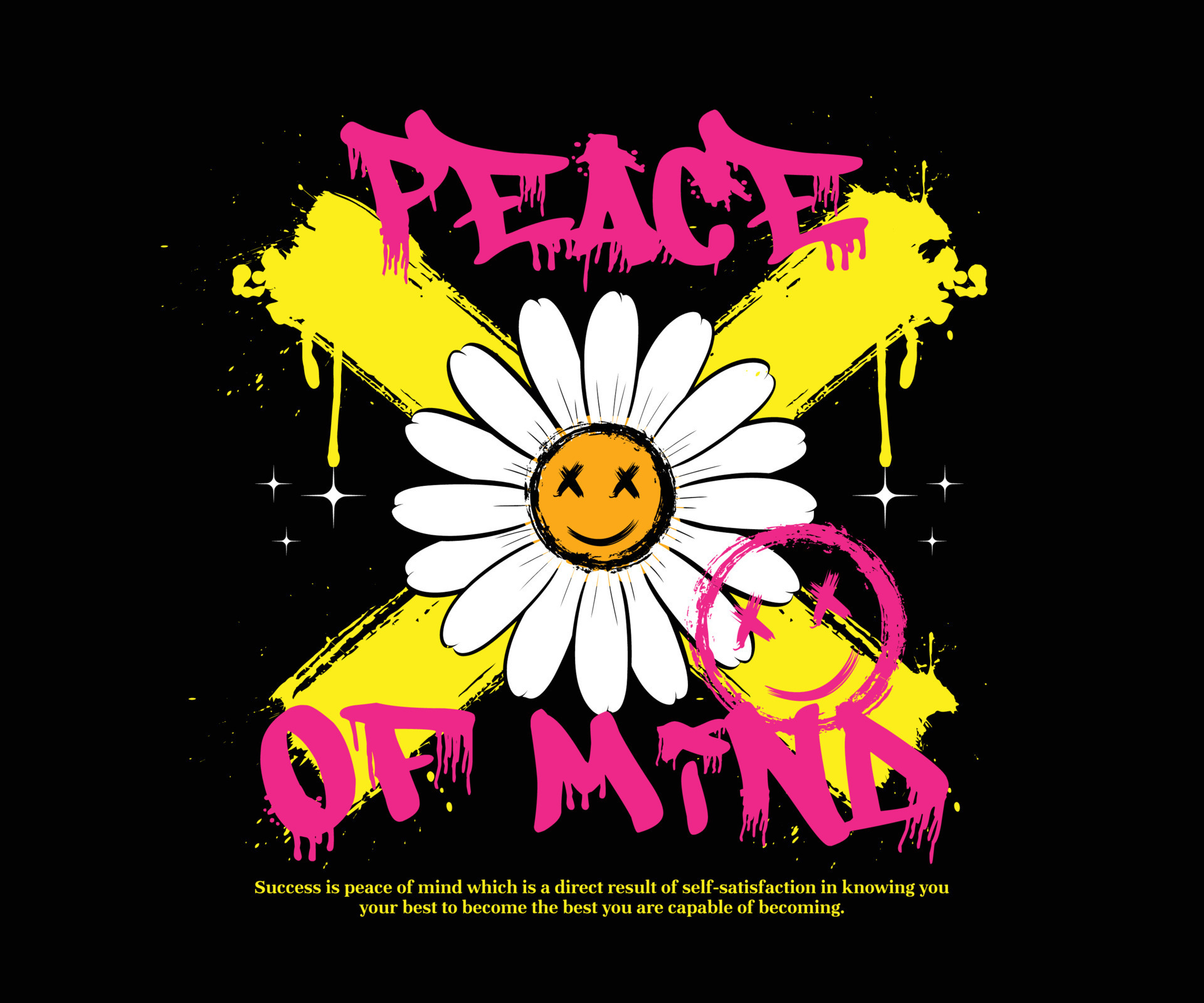This square image features a stark black background with a central dripping, painted yellow "X." Above the "X" in jagged, drippy, all-caps text is the word "PEACE," while below the "X" it reads "OF MIND." In the center of the "X," a flower with white petals, a yellow center, and black "X"s for eyes and a smiley face adds a whimsical touch. On the right of the flower, above the "ND" in "MIND," is a pink circle with "X"s for eyes and a smiley face. Flanking the flower are white diamonds of varying shapes and sizes. Underneath the main elements, in yellow text spanning two lines, it says: "Success is peace of mind, which is a direct result of self-satisfaction in knowing you're doing your best to become the best you are capable of becoming." Small stars are scattered at the base of the paint drips, enhancing the graffiti-like aesthetic of the artwork.